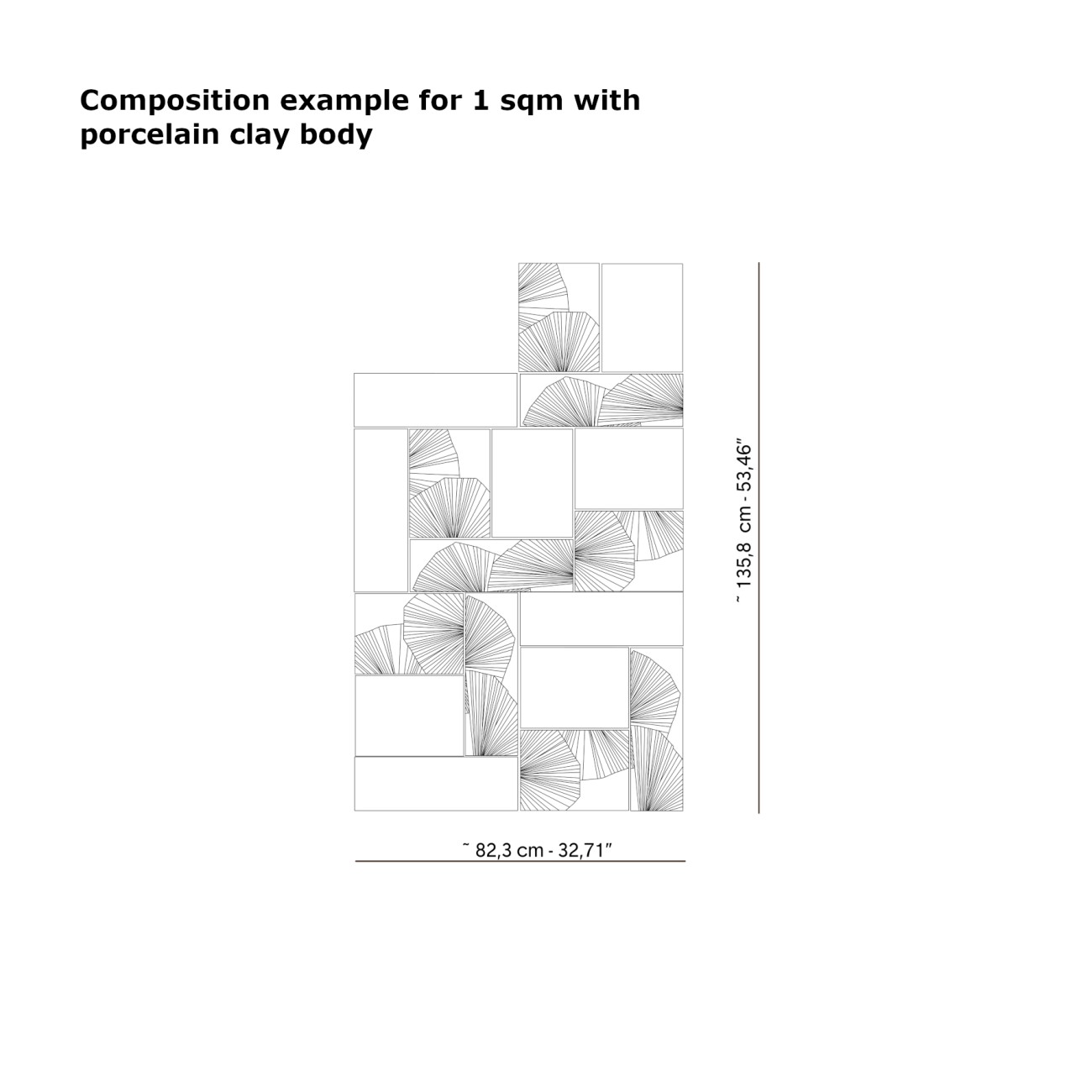This image is a detailed rendering from a textbook, featuring a diagram labeled in bold Verdana font at the top: "composition example for one square meter with porcelain clay body." The illustration, which measures 82.3 centimeters in width and 135.8 centimeters in height, consists of a series of linked rectangles. Some of these rectangles contain finely sketched fan patterns or other intricate designs. The diagram resembles a puzzle, where these uniquely shaped and meticulously pencil-drawn components could be arranged to form a cohesive composition. Solid lines border the bottom and right sides, further emphasizing the structured layout of this composition example.